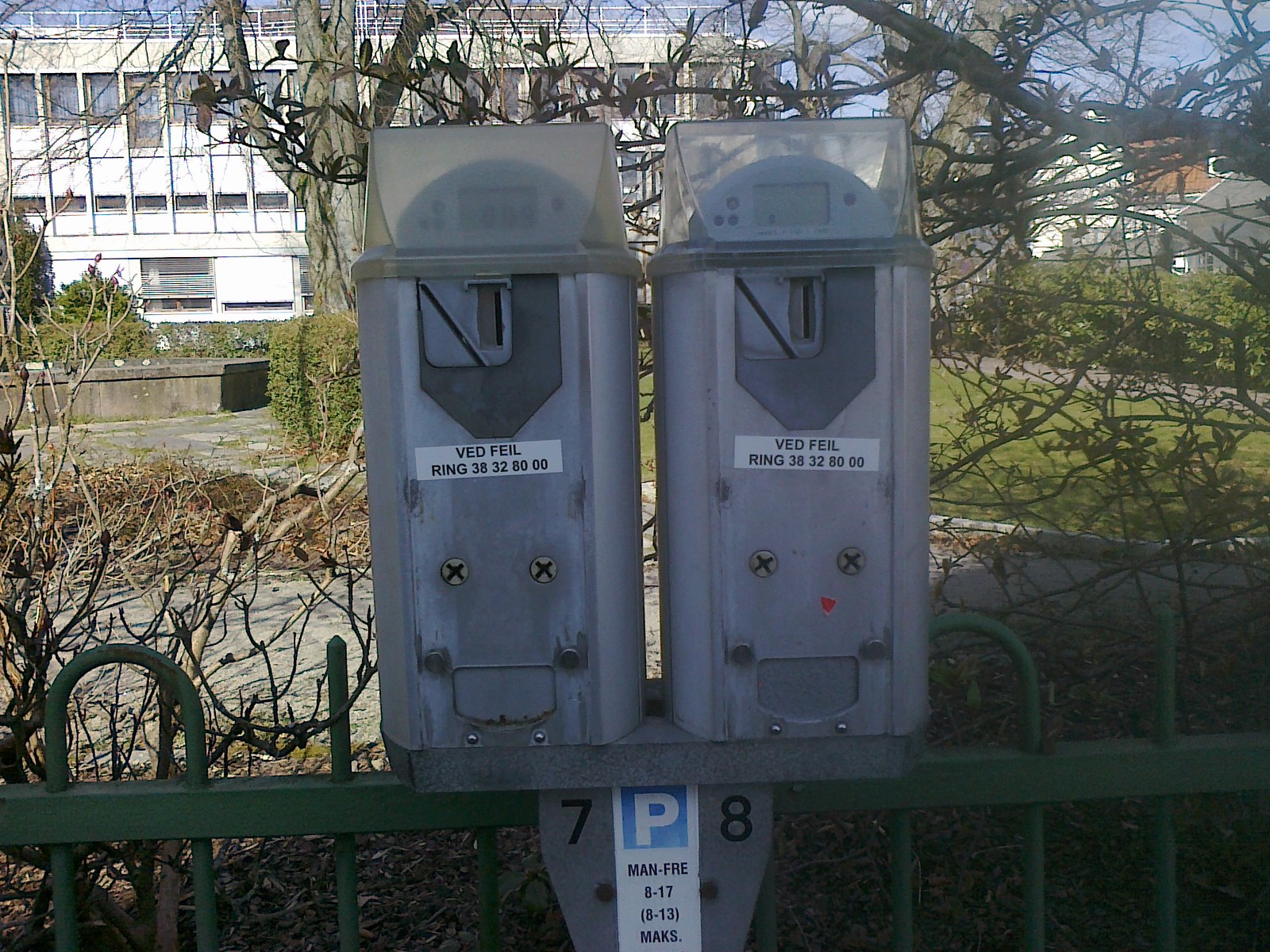This image features two tall, gray-colored steel parking meters mounted on a gray base atop a green wrought iron fence. The parking meters have rectangular shapes with sleek, modern designs. Each meter has a clear plastic cap at the top, protecting small LED readout screens. Below the screens, there is a coin slot designed for inserting quarters. A white sticker on the front middle of the meters reads, "Venn Field, ring 38-32-80-00," which suggests these meters are likely located in a foreign country. Towards the bottom, the meters are secured with two large bolts, and there is a small flappy door for retrieving change. Below the meters, there is a sign featuring a large "P" with "MAN-FRE" underneath, followed by "8-17," "(8-13)," and "M-A-K-S" at the bottom. In the background, the scene includes green grass on the right-hand side, a patch of gray pavement on the left, a small portion of brown, and the silhouette of a white building in the left-hand corner.